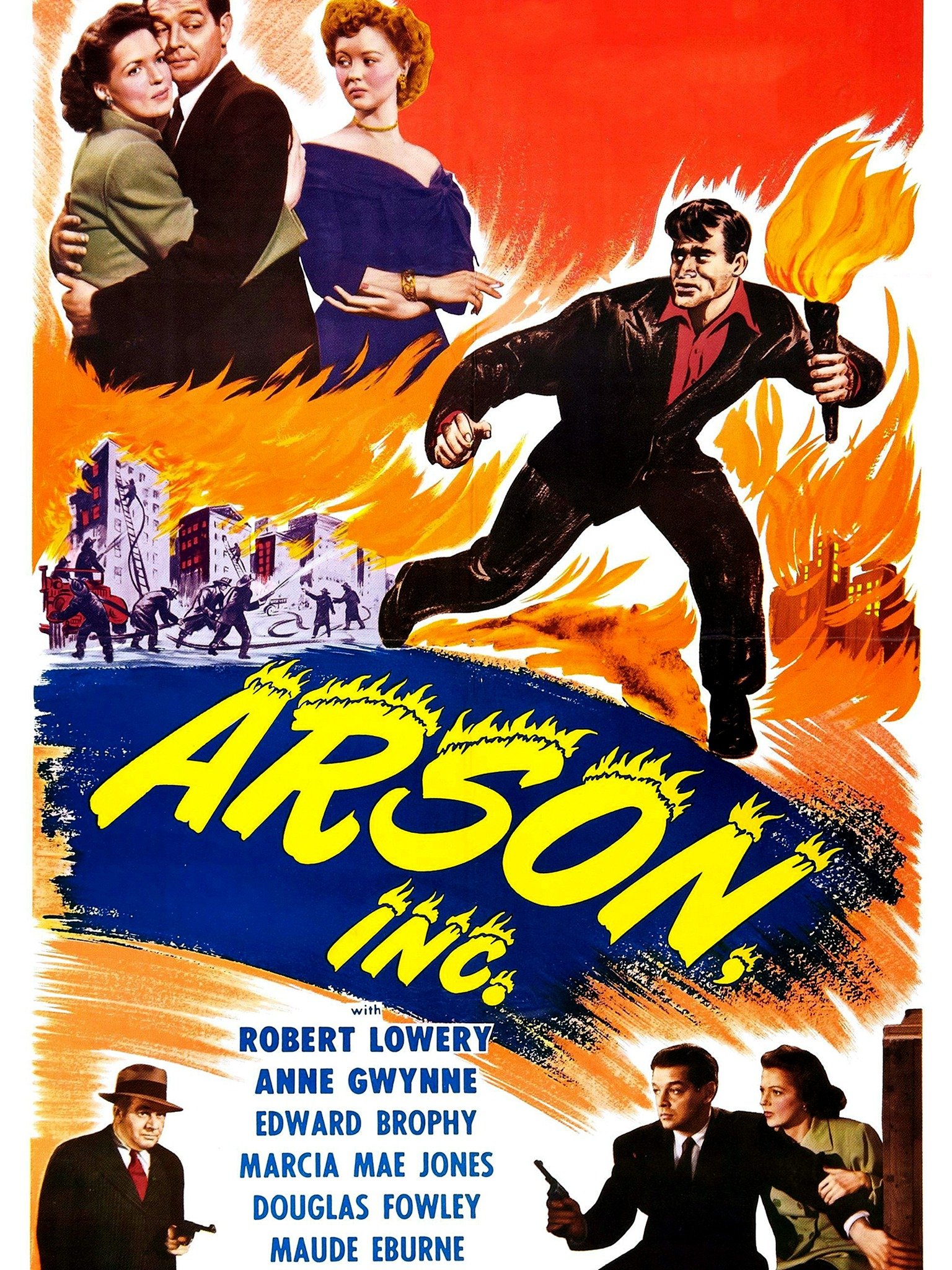The image is a detailed and vibrant poster for a film titled "Arson Inc." The predominant background color is red, contributing to the dramatic flair of the poster. In the top right corner, there's an evocative scene featuring a man in a black suit and a woman in a light brown jacket embracing, while another woman in a blue dress looks on disapprovingly. Below them, cartoon flames flicker, hinting at a theme of fire and danger.

To the right, a man in a black jacket, black pants, and a red shirt is depicted running with a flaming torch, his expression suspicious as he flees the scene. Behind him, firefighters are battling a blaze at a building, emphasizing the film's arson-related plot.

A blue banner at the bottom prominently displays the title "Arson Inc." in bold yellow text. Below this, the names of the cast members are listed in blue text: Robert Lowry, Anne Gwynne, Edward Brophy, Marcia May Jones, Douglas Fowley, and Maude Eburne. Additional small cutout scenes of the actors are scattered throughout, adding depth and intrigue to this vintage movie poster.